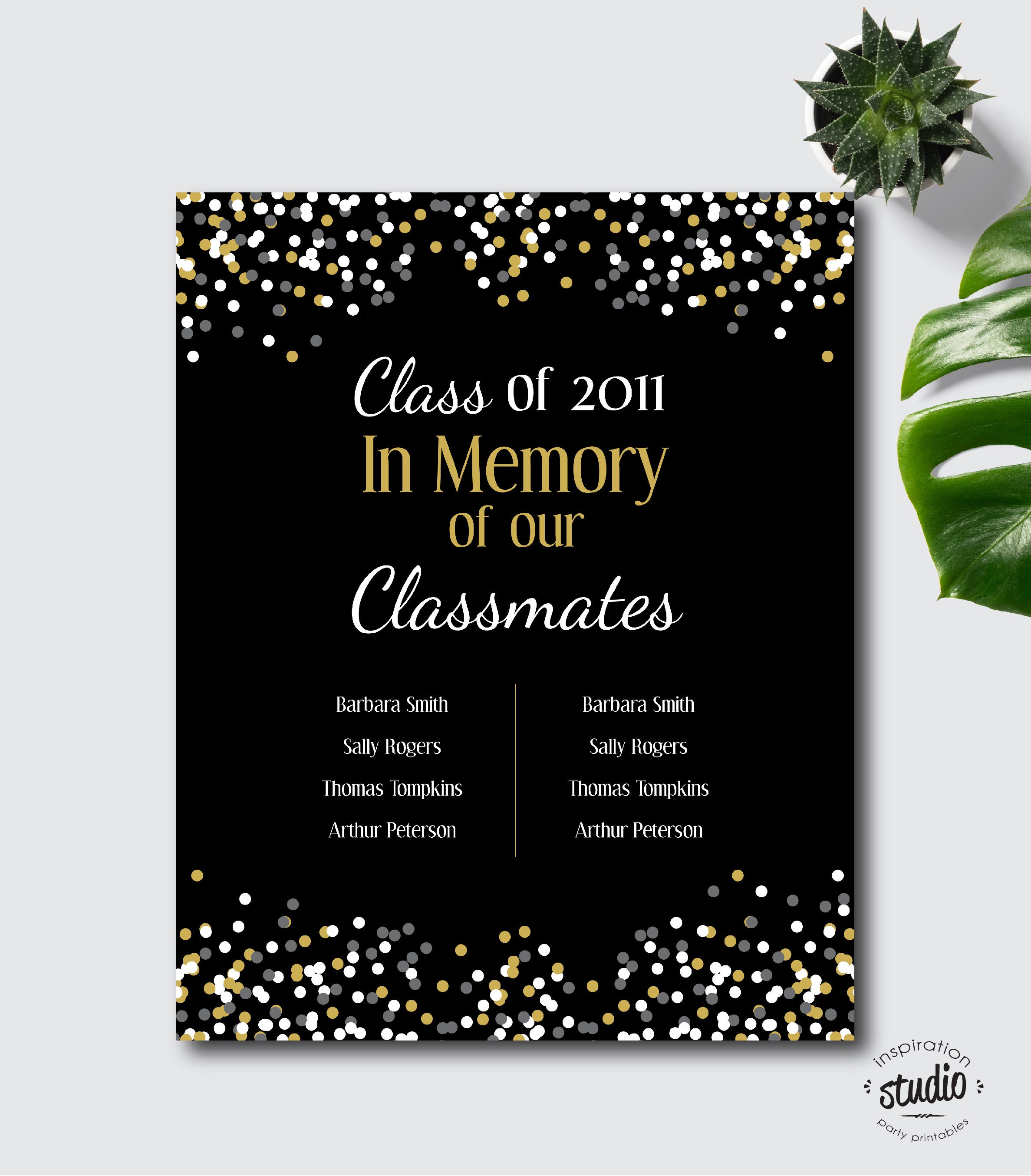The image showcases a downloadable template designed for adding personal images, often used for product photos. It features a sleek gray background adorned with a monstera leaf and a succulent plant for visual interest. Dominating the center is a black poster trimmed with black, gold, gray, and white confetti-like designs along the top and bottom edges. The poster, which is presumably meant for a class reunion, reads "Class of 2011" in white and "In Memory of Our" in gold, followed by "Classmates" in white. Below this heading, eight names are listed in two columns, each repeating Barbara Smith, Sally Rogers, Thomas Tompkins, and Arthur Peterson. The poster appears to honor deceased classmates. In the bottom right corner of the image, the watermark "Inspiration Studios Party Printables" appears in black lettering, ensuring credit to the creator.